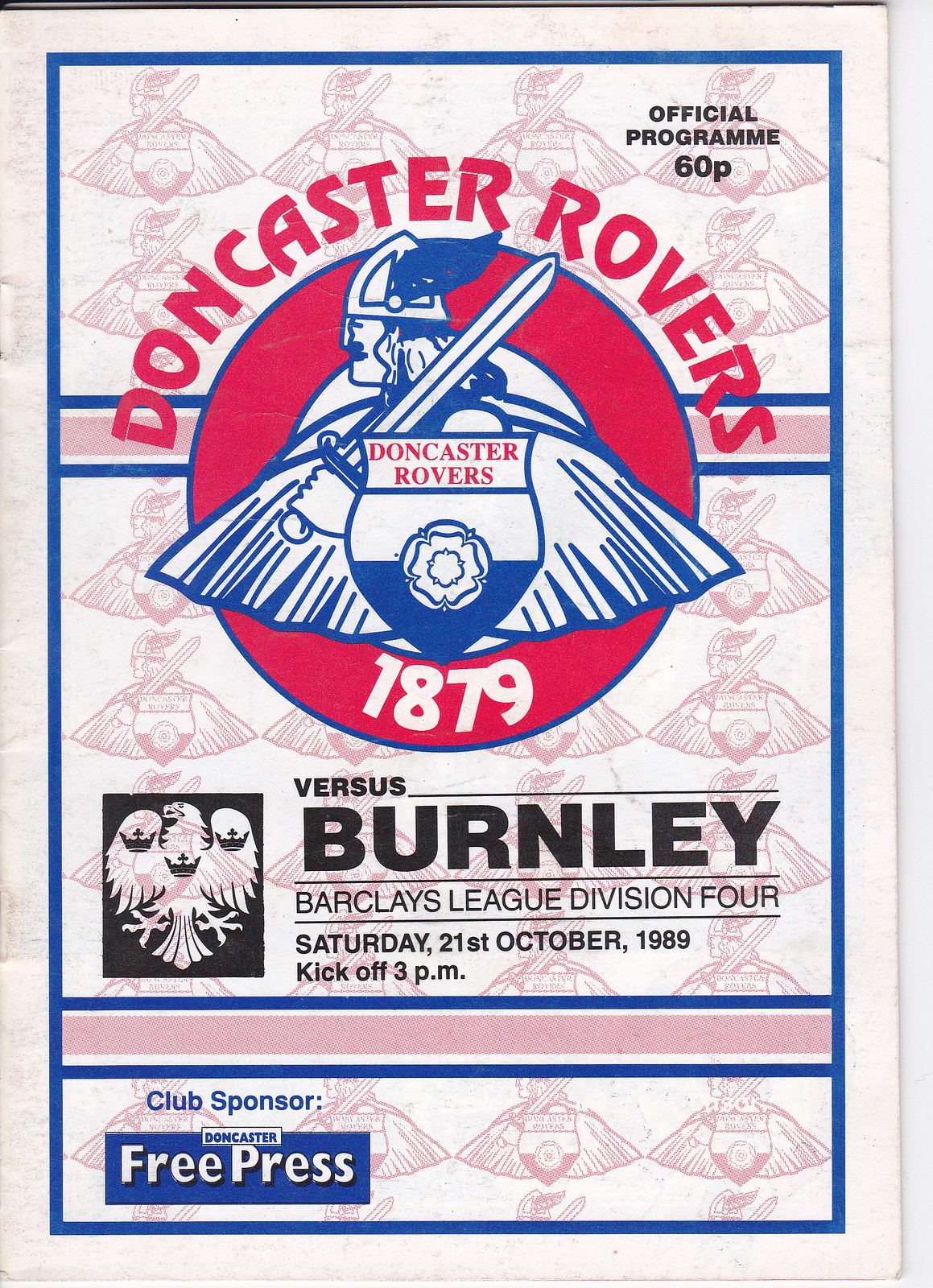The poster, framed in blue, is predominantly white and features an elaborate design that includes multiple logos in the background. At the top center, "Doncaster Rovers" is prominently displayed in red text, and just below it is a circular red outline with a blue inner border. The main logo within this circle showcases the side view of a knight-like warrior holding a sword and adorned with a helmet featuring a feather, accompanied by a shield bearing the words "Doncaster Rovers." Alongside the emblem, in white text, is the year '1879.' To the top right in black text, the words "Official Program 60p" are visible.

The poster also displays event information, which reads: "Versus Burnley, Barclays League Division 4," followed by the date and time "Saturday, 21st October 1989, kick-off 3 p.m." Additionally, there's a notable black logo on the left of an eagle, carrying three crowns displayed on its wings and chest. The bottom section of the poster includes the club sponsor "Doncaster Free Press" and features a distinctive pink strip.